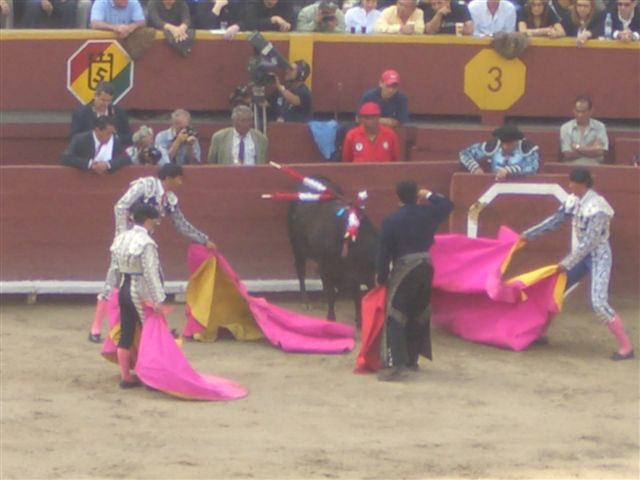The image depicts a live bullfight event set in a Spanish arena with sandy grounds. The arena is surrounded by vibrant red and yellow stands packed with spectators attentively watching the spectacle behind a sturdy fence. In a more distant layer, another fence is visible with a man capturing the moment on his camera, positioned to photograph the engaging crowd and show. A red, yellow, and green striped sign is noticeable in the background.

At the forefront of the scene are three matadors outfitted in striking white attire adorned with intricate bedazzlements, accompanied by pink socks and black loafers. Each matador brandishes a vivid pink cape with a yellow underside towards an imposing black bull stationed centrally in the ring. Alongside them stands a fourth man clad in all black, wielding a red cape and assuming a poised stance with an arm raised in salute. The bull, highlighted in the middle of this dynamic arrangement, bears three spears in its back and is also seen with a red and white striped object, resembling a pole, attached to it.

The spectators' expressions and the diligent activity of multiple photographers - including an older couple with cameras, a suited gentleman, a man in a red shirt and cap, a man with a video camera, and another individual with a tan shirt and crossed arms - add layers of depth to the image, encapsulating the intense atmosphere and cultural richness of an authentic bullfighting event.